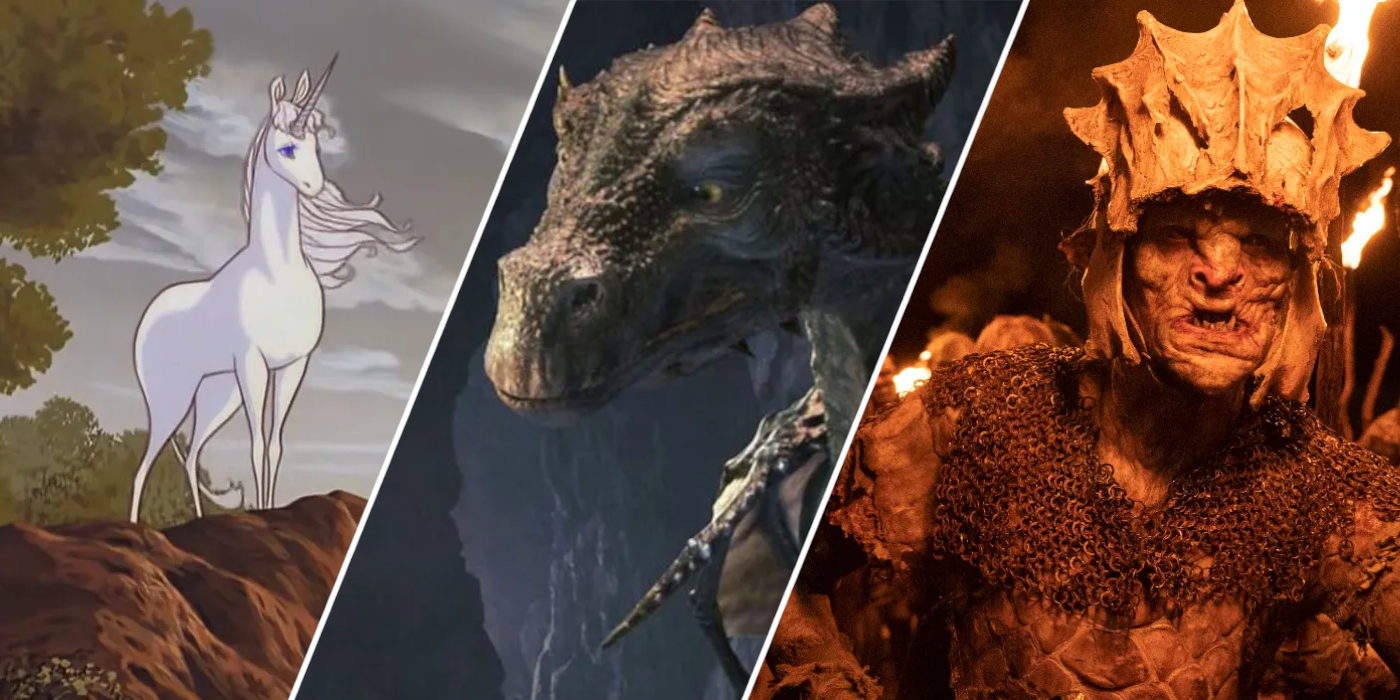The image is a collage of three distinct scenes, each separated by diagonal white lines. On the far left, there's a cartoonish depiction of a majestic white unicorn. It stands proudly on a brown rocky hill, surrounded by distant trees and set against a backdrop of gray, cloudy skies. The unicorn has a long, flowing white mane, blue eyes with a hint of purple, and a spiral-shaped, pointy horn on its forehead.

The middle section features a dragon, seemingly from a TV show or movie, situated in a dark, cave-like environment. This dragon is predominantly brown with scaly, lumpy skin and four horns protruding from its head. Its yellowish eyes with black pupils give it an innocent appearance, despite its formidable features.

On the far right, the image showcases a monstrous creature resembling an orc or goblin in a dimly lit cave with flickering torches casting an amber glow. This grotesque figure has a deformed face with a crooked nose and jagged teeth, some protruding from an underbite. The skin appears scaly and clammy. Adorned in worn-out rusty chainmail, the creature also wears a helmet made from the bone of some ancient beast, complete with menacing horns. The overall appearance conveys a sense of medieval and mythical horror.